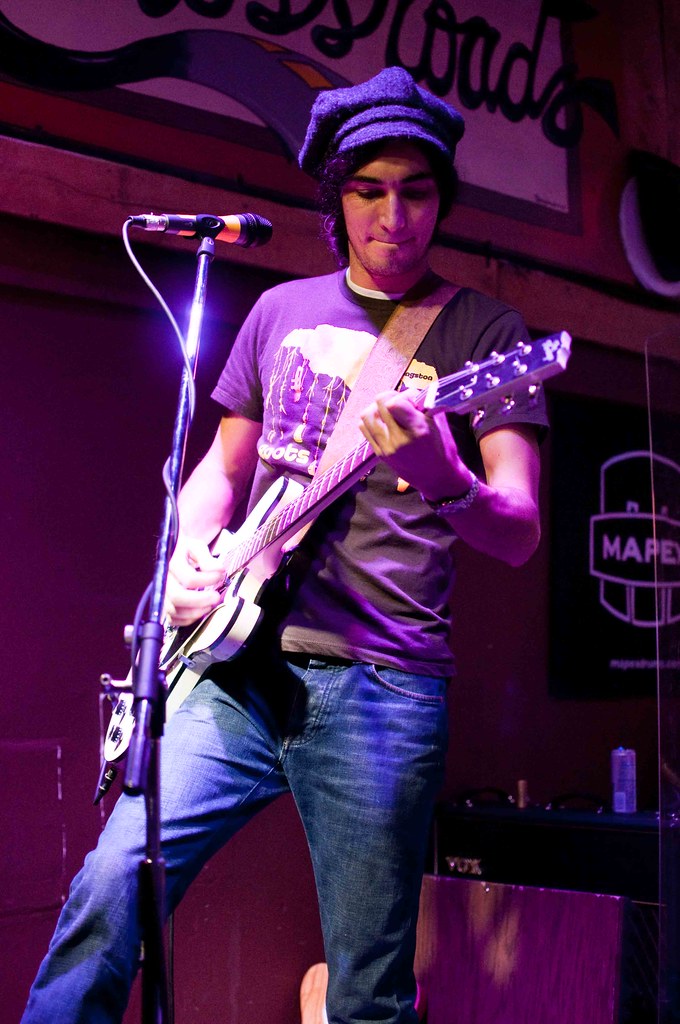In the photograph, a rock musician stands on a stage, captured mid-performance. A prominent black microphone stand with a reflective metallic material and a black rubber-like wire wrapping is positioned in the forefront. This stand supports a yellow and black microphone, angled towards the musician. The man, attired in blue jeans and a dark brown graphic T-shirt adorned with a stylized white tree with spreading roots or vines, is also wearing a distinctive gray English cap. Draped across his shoulder is a light brown leather guitar strap holding a white electric guitar with black trimming and a wood-colored neck. Behind him, the stage background features a black sign with white writing that says "MAPE,” a speaker with an aluminum can on top, and the edge of another guitar, hinting at a rich musical environment. The musician appears to be in the midst of strumming his guitar, possibly accompanying other instruments, as he is not currently engaged with the microphone.